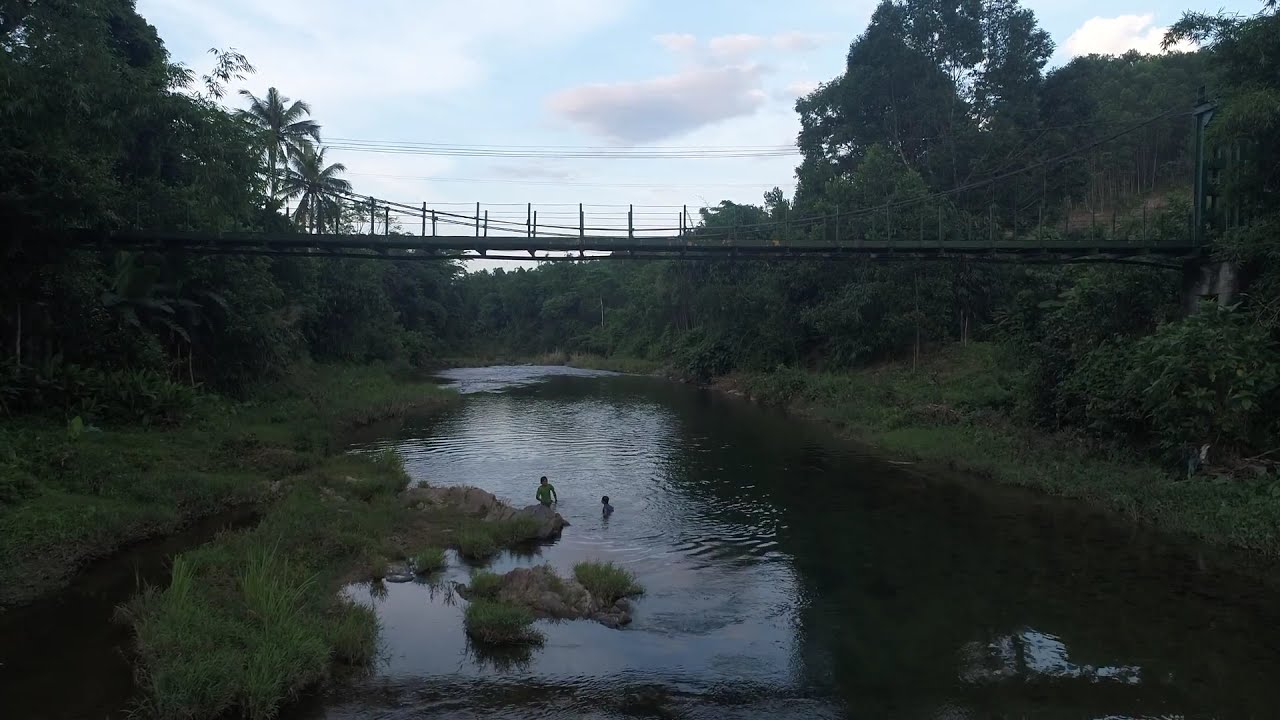This rectangular photograph captures a scenic, tropical river landscape at dusk, characterized by its calm, dark waters running through the center of the composition. A bridge, made of a combination of metal, wire, and wood, spans horizontally across the river, approximately 50 feet above the surface. The bridge features metal bars and cables forming a barrier on both sides, with suspension cables stretching from the left corner, dipping towards the center, and attaching to a bar on the right. Above the bridge, a set of power lines can be seen crossing the sky.

The river itself is flanked by lush, verdant greenery, including grass along the banks and densely packed trees, some of which are tall tropical palm trees and others with thick, impenetrable foliage. A small almost island-like area juts into the river from one side. Two children are swimming in the water, their distant profiles just visible; one child stands a bit taller with arms hanging by their sides, while the other is slightly shorter, near the center of the river.

The sky above is a light blue adorned with a mix of dark gray and white low-flying clouds, creating a serene but somewhat shadowy ambiance indicative of dusk. Light reflections and ripples can be observed on the right side of the river, where the water is tinged green and appears slightly lighter compared to the darker left side. Overall, the photograph beautifully encapsulates the tranquil yet lively essence of a tropical evening by the river.